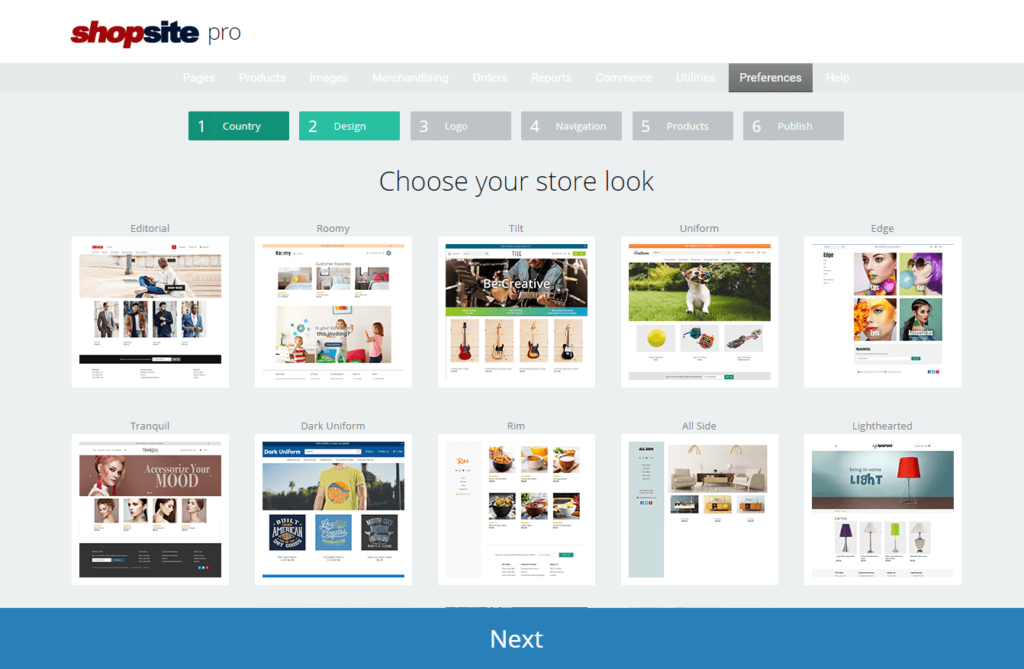The image is a horizontally oriented screenshot from a website accessible via computer or smart device. The interface belongs to ShopSite Pro, as indicated by the prominent label at the top against a white background. Below it, a dark gray navigation strip displays a series of menu options in white font: Pages, Products, Images, Merchandising, Orders, Reports, Commerce, Utilities, Preferences (highlighted in dark gray), and Help. Directly below the navigation strip, the background transitions to a lighter gray.

In this lighter gray section, green text labels indicate "Country," followed by a lighter green "Design," and then a return to gray for item labels such as "Logo for Navigation," "Products," and "Publish."

Below this is a black header reading "Choose Your Store Look," under which are two rows of visual options for store themes. The top row features Editorial, Roomy, Tilt, Uniform, and Edge, while the bottom row showcases Tranquil, Dark, Uniform Rim, All-Side, and Lighthearted. Each option includes a thumbnail image to preview its appearance.

At the very bottom of the image, a blue bar with the text "Next" indicates a progression button for continuing to the next step.